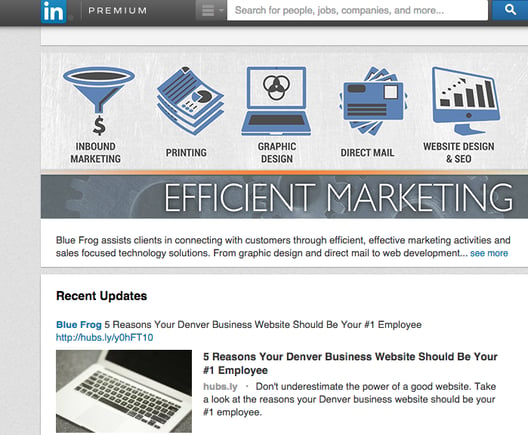The image features the LinkedIn logo prominently displayed in the upper left-hand corner, set against a gray bar that spans the top of the image. To the right of the LinkedIn logo, the word "Premium" is visible, followed by a search bar which includes placeholder text that reads: "Search for people, jobs, companies, and more."

Beneath this top section, there's a horizontal row of categorized options, each accompanied by an icon. The categories listed are: "Inbound Marketing," "Printing," "Graphic Design," "Direct Mail," "Website Design," and "SEO."

Below these categories is another gray bar, inscribed with the phrase "Efficient Marketing," stretching across the width of the webpage. Following this, a white bar appears, containing two lines of text which are not specified.

At the very bottom of the image, a partially cut-off white box labeled "Recent Updates" is visible, indicating the start of a section featuring the most current information or activities.